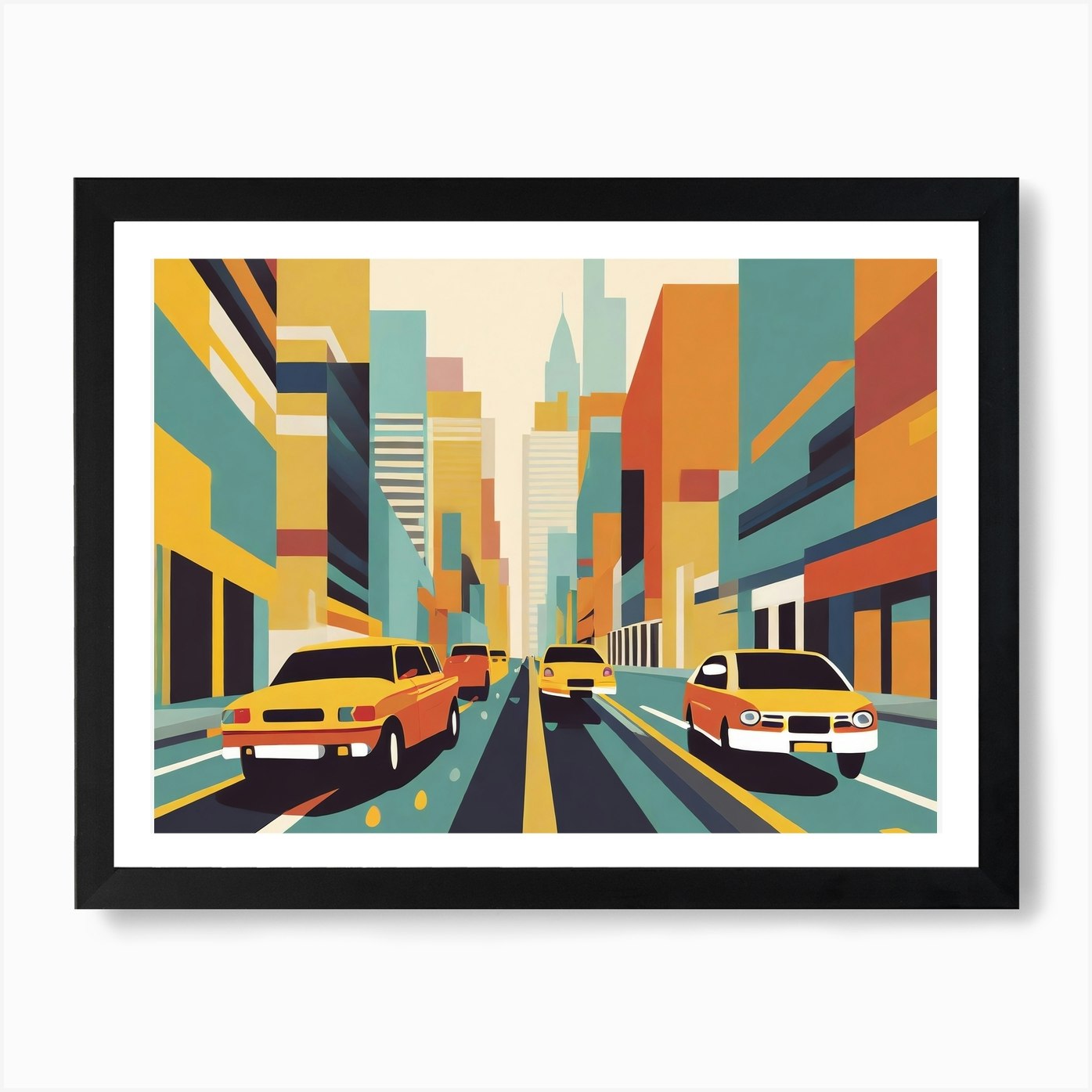The image showcases a detailed digital painting with a solid black frame, resembling a piece of artwork set against a white background. The scene depicts a bustling city street filled with five yellow and orange cars driving both towards and away from the viewer on a two-lane road. The street itself is rendered in a dark blue or teal shade with yellow and white lines marking it. Tall skyscrapers line both sides of the street, adorned with bands of posterized colors including orange, blue, yellow, green, and brown, giving the buildings a blocky and stylized appearance. These buildings are likely meant to represent windows in a simplified form. In the distant background, additional large skyscrapers rise up, potentially including iconic structures such as the Empire State Building, hinting that the city could be New York. The sky visible between the skyscrapers is an unnatural white cream color, adding to the painting's digital and somewhat abstract feel. Despite the subdued and constrained color palette, the image exudes a vibrant urban atmosphere.